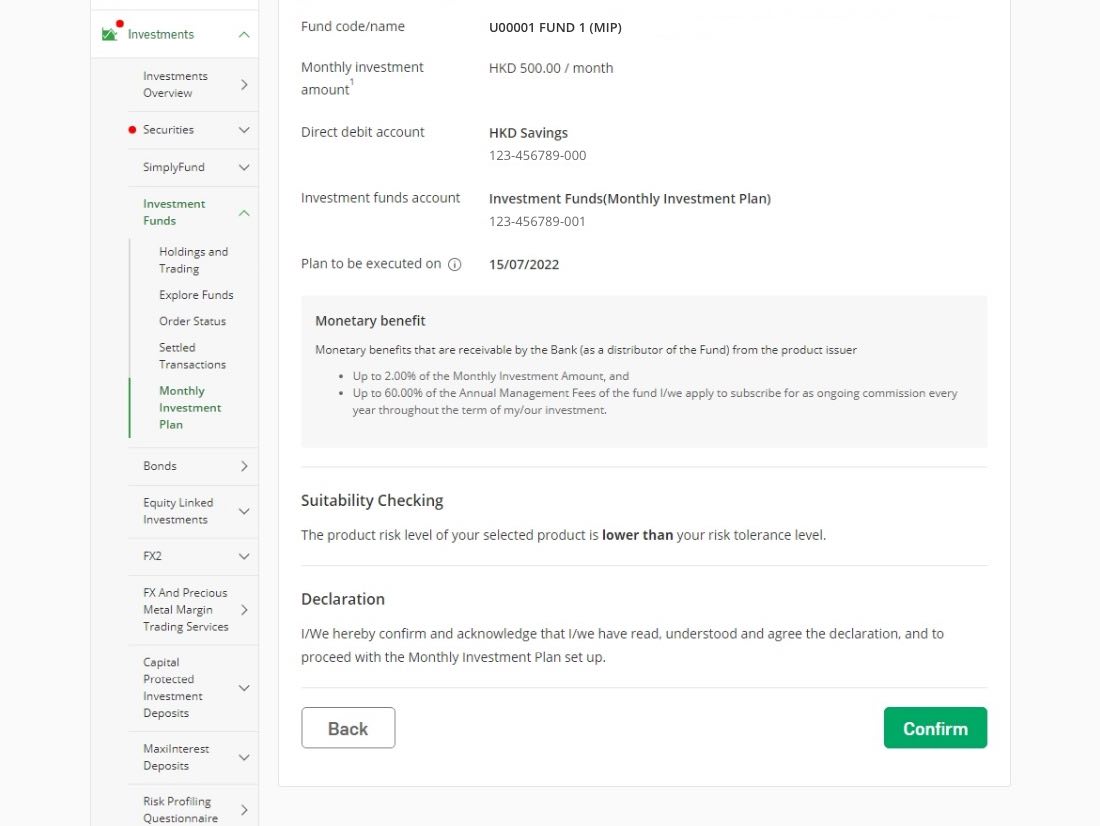This image depicts the investments section of a financial website with a dual-tone background. The left side features a light gray color with a vertical bar extending from the top to the bottom, while the right side has a white background.

In the top left corner, the header reads "Investments," accompanied by a green icon or logo with a red circle next to it. Directly beneath this header, there are multiple tabs for navigation, including:
- Investments Overview
- Securities
- Simple Fund
- Investment Funds
- Holdings and Tradings
- Explore Funds
- Order Status
- Settled Transactions
- Monthly Investment Plans
- Bonds
- Equity-Linked Investments
- FX2
- FX and Precious Metal Margin Trading Services
- Capital-Protected Investment Deposits
- Interest Deposits
- Risk Profiling Questionnaire

On the right side of the page, detailed account information is displayed. This includes sections for the investment amount, the planned execution date, monetary benefits, suitability checking, and declarations. At the bottom of the page, there are two buttons for user interaction: "Back" and "Confirm."

The overall layout is designed to provide a comprehensive overview of various investment options and account details in a structured and user-friendly manner.